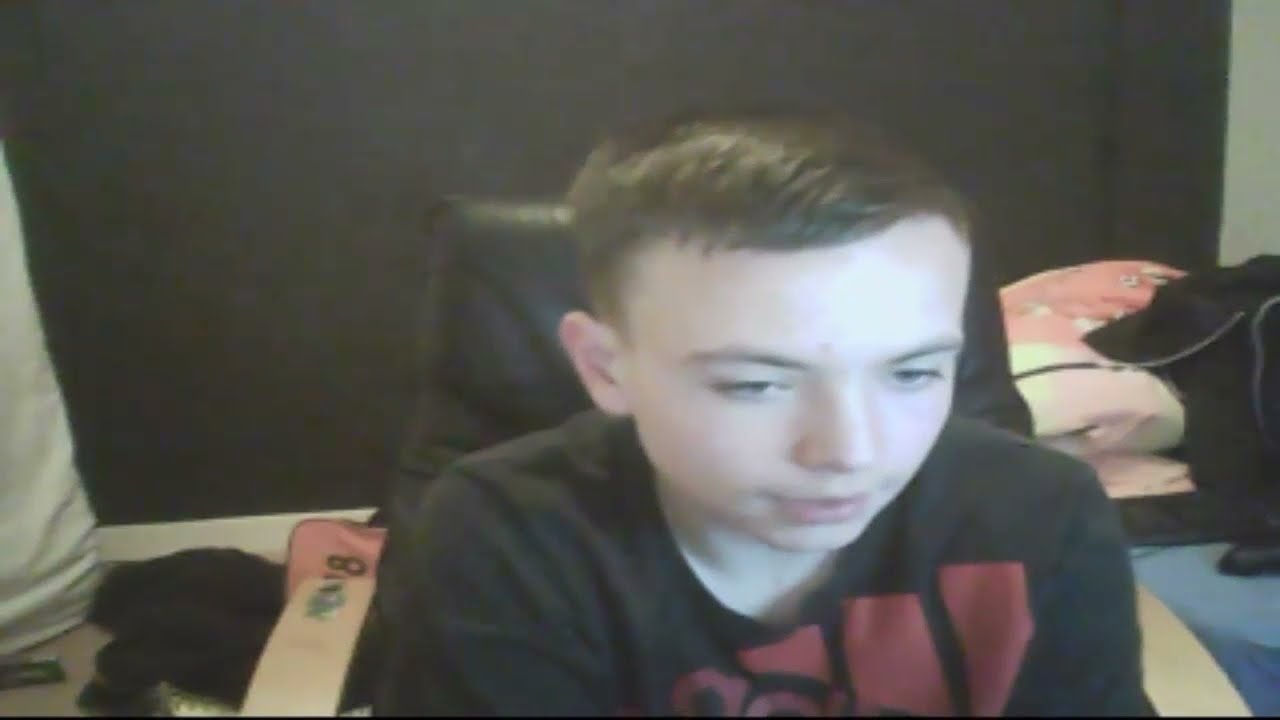The image features a young boy, likely in his early teens, with short, closely cropped dark hair. He has a round face and a light skin complexion, displaying an expression of intense interest as he looks slightly downward, possibly focusing on a laptop or monitor. The boy is seated in a black leather chair, wearing a black short-sleeve Adidas t-shirt with a prominent red logo on the front. The background includes a black wall and, to the right, a white cushion or chair. The image has a webcam-quality feel, suggesting it might be a screenshot from a video or livestream, capturing a moment where the boy is deeply engaged with whatever is on his screen.